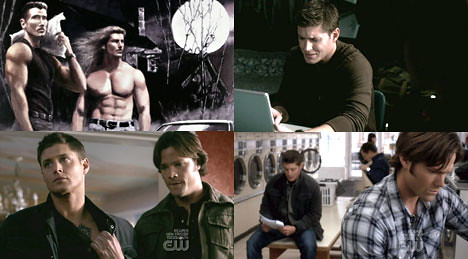The image is likely a screen capture from the show "Supernatural," featuring four smaller pictures within it. The top left picture shows two muscular men, one on the right with long hair and no shirt, resembling the model Fabio, and the other on the left with short brown hair, wearing a black sleeveless shirt. The background includes a haunting scene with a large white moon, barren trees, and a spooky house. The top right picture captures a man in a brown long-sleeve shirt or hoodie, appearing frustrated while working on a silver laptop, seated on a green plastic chair. Below this, in the bottom left image, two men are present: one is tugging at the collar of his shirt, revealing a tattoo on his chest, while wearing a brown jacket; the other stands beside him wearing an olive green jacket. There is also a CW network watermark in this segment. Lastly, the bottom right picture shows two men in a laundromat, one seated in front of a laundry machine, with more people visible in the background.